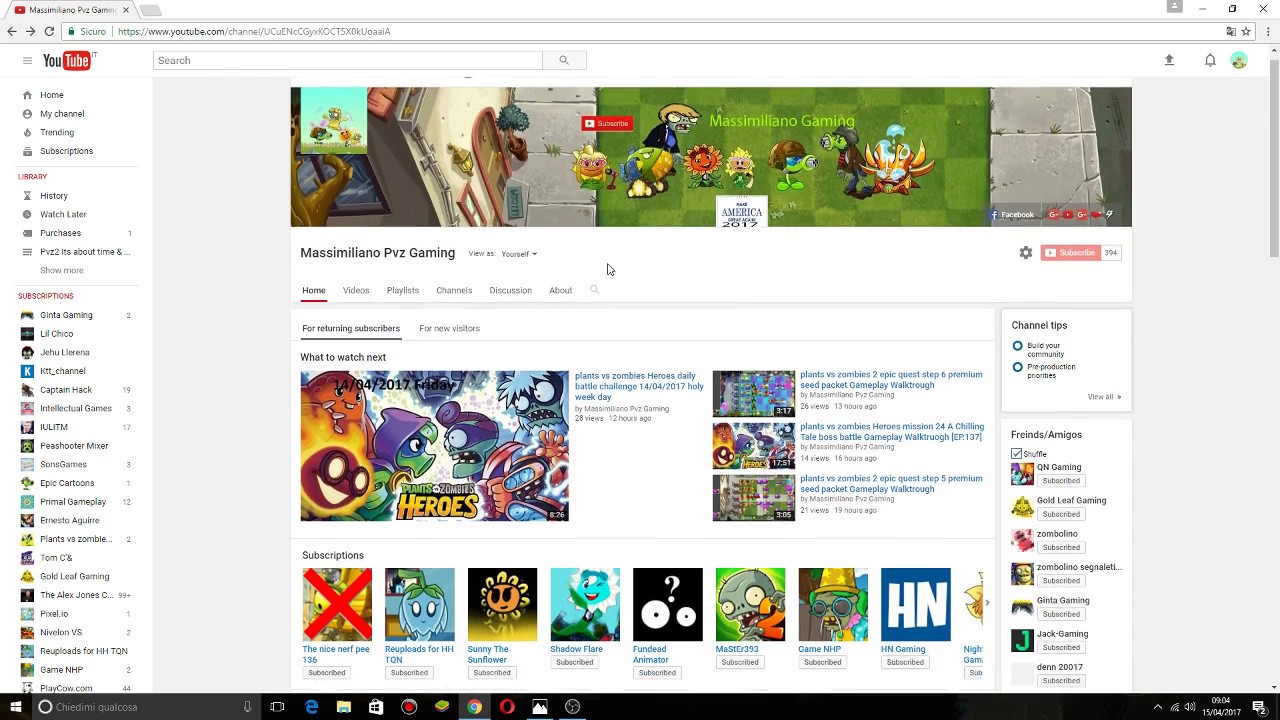The image is a detailed screenshot of a YouTube page displayed in a browser window. Prominently featured in the upper left corner is the recognizable YouTube logo. Just to the right, the URL bar is visible, with the search bar positioned at the top center of the YouTube interface. On the left-hand side, a vertical menu lists various navigational options such as Home, My Channel, Trending, Subscriptions, Library, History, Watch Later, and Purchases. Below these options, a list of the user’s subscriptions is displayed, showcasing several channels.

The main focus of the screenshot is the YouTube channel page for "Messimilano PVZ Gaming." At the top of this page is a banner image that appears to be a screenshot from a game, featuring charming cartoon creatures. Directly below the banner, tabs for Home, Videos, Playlists, Discussion, and About are visible, with the Home tab currently selected. The body of the page displays various video thumbnails, representing the channel’s content and subscriptions. The overall layout is typical of a YouTube channel home page, providing easy access to the creator's uploaded content and interactive features.